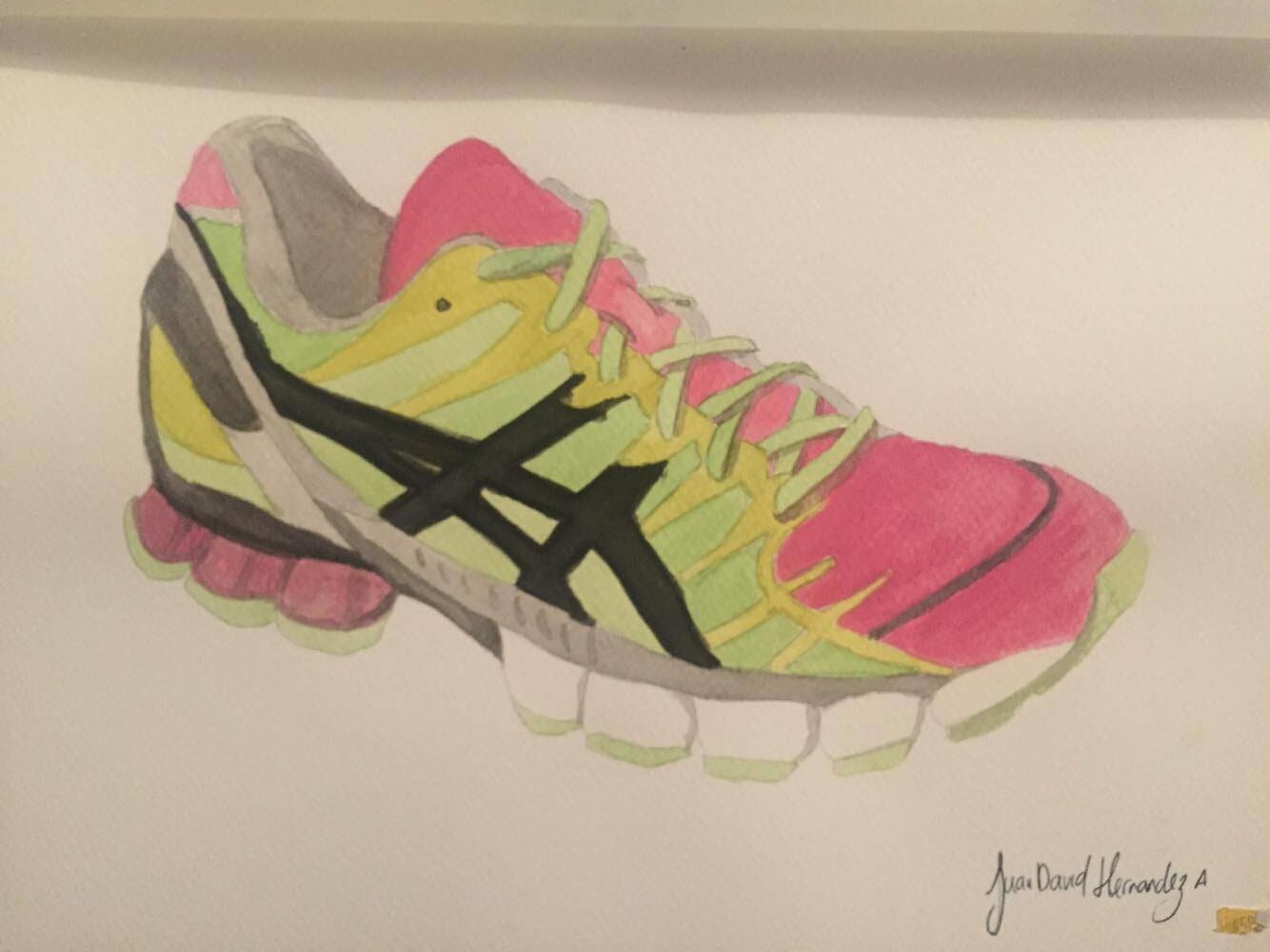The image depicts a vibrant, detailed drawing of an athletic sneaker, seemingly created with colored pencils. The front of the shoe is predominantly hot pink, including the tongue, complemented by vivid lime green shoelaces that cross intricately up the shoe. The side of the sneaker features light green as its primary color, accented with yellow lines and thick black trim. The heel and the grips on the bottom of the sole are dual-colored with pink and lime green, while the front part of the sole is white. Inside the shoe, the lining appears to be gray. The sneaker’s dynamic design is punctuated by a signature in the bottom right-hand corner, which reads "Juan David Hernandez," indicating the likely artist. The shoe, facing the right side of the image, gives off an impression of being a running shoe, full of vibrant energy and eye-catching detail.